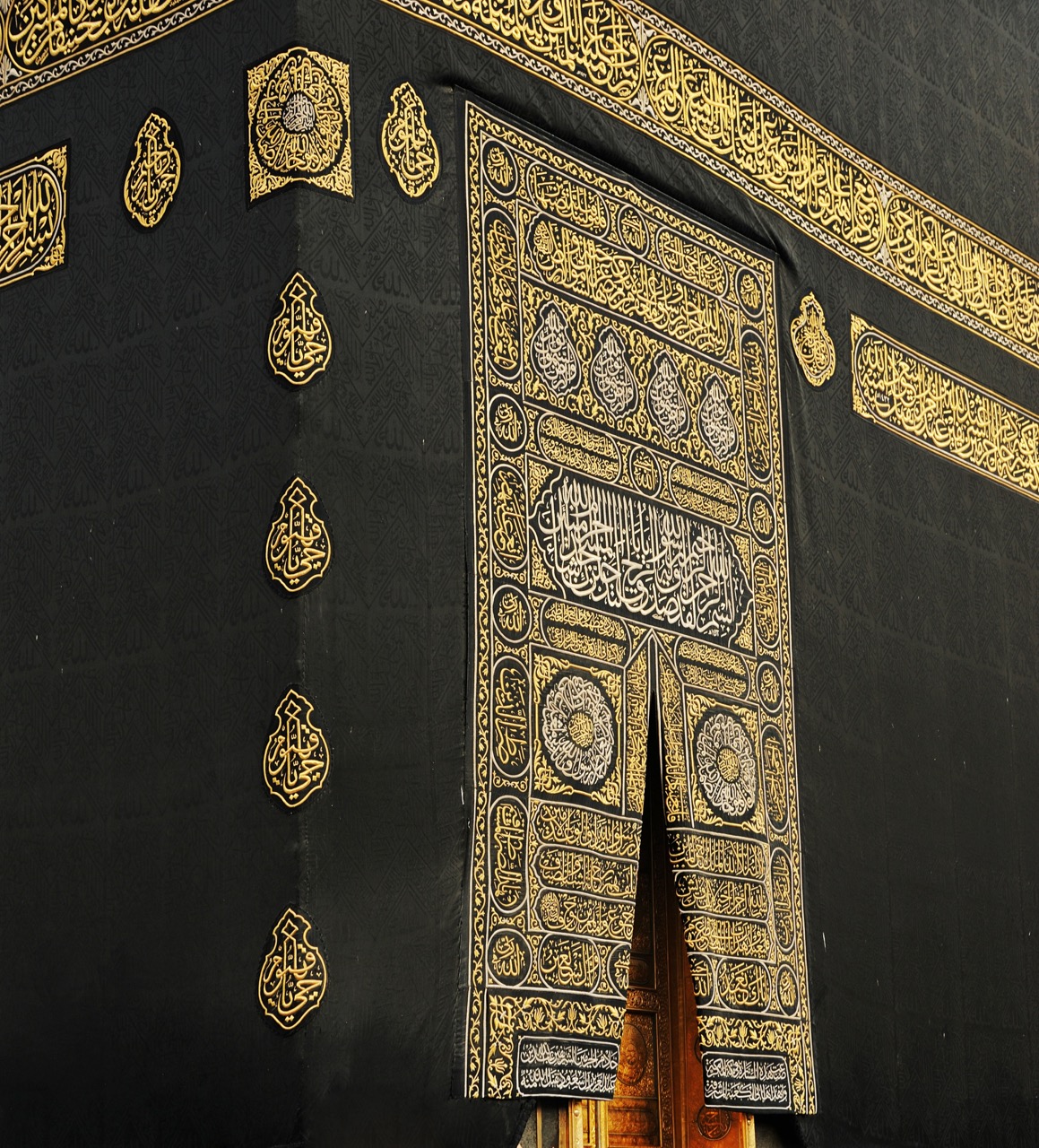The image showcases a tall, rectangular woven tapestry with a dark, black fabric decorated with intricate tile-shaped patterns. This tapestry, possibly hung in a museum or a grand building, appears to drape over a wooden structure, subtly visible just to the right of the center near the bottom. At the top right corner, a diagonal golden woven design runs toward the upper edge of the tapestry, vanishing at the top and reappearing in the top left corner, as if extending over a corner of the structure. The tapestry is adorned with Islamic-inspired patterns and features contrasting golden bands and squares. These golden patterns give the impression of a curtain covering a rectangular section, potentially resembling a door, which also seems to have golden embellishments. Additionally, on the left side of this dark curtain, there are symbols arranged in four horizontal and vertical lines. The fabric splits apart at the bottom, enhancing the decorative allure of the scene.